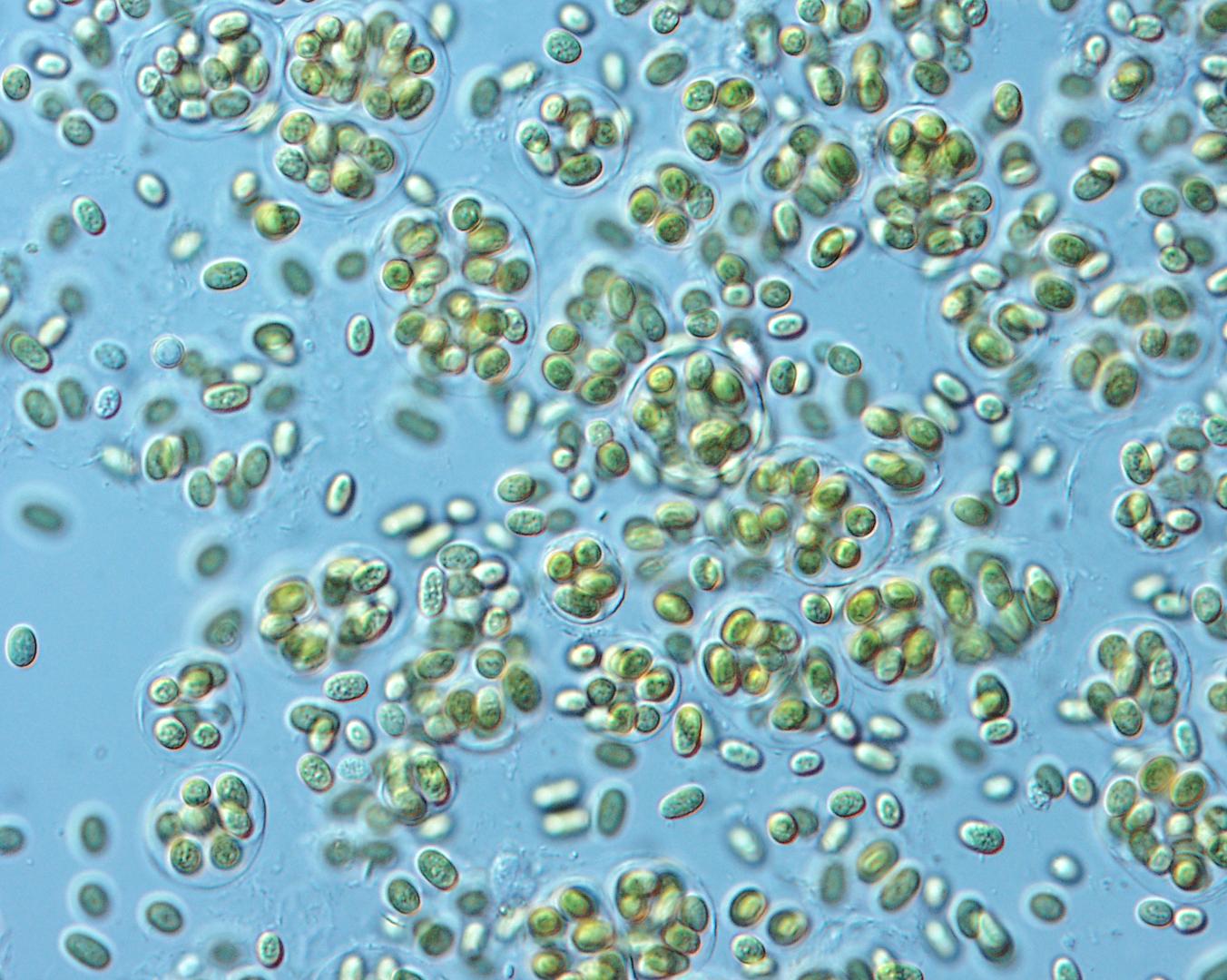This is a highly detailed microscope image displaying an abundance of circular and oval-shaped cells, set against a blue background. The cells exhibit varying colors, predominantly green, white, and blue. Some cells appear as individual entities with clearer, bluish tones, while others cluster within distinct round borders, showcasing a green hue suggestive of plant cells. Among these clusters, several show signs of cell division. Additionally, a few darker, grayish cells are present, resembling shadows. Notably, the clusters with clear circular borders, though fewer, are concentrated particularly at the center and more towards the left side of the image. Overall, the intricate mosaic of hundreds of cells, both individual and grouped, dominates the image.